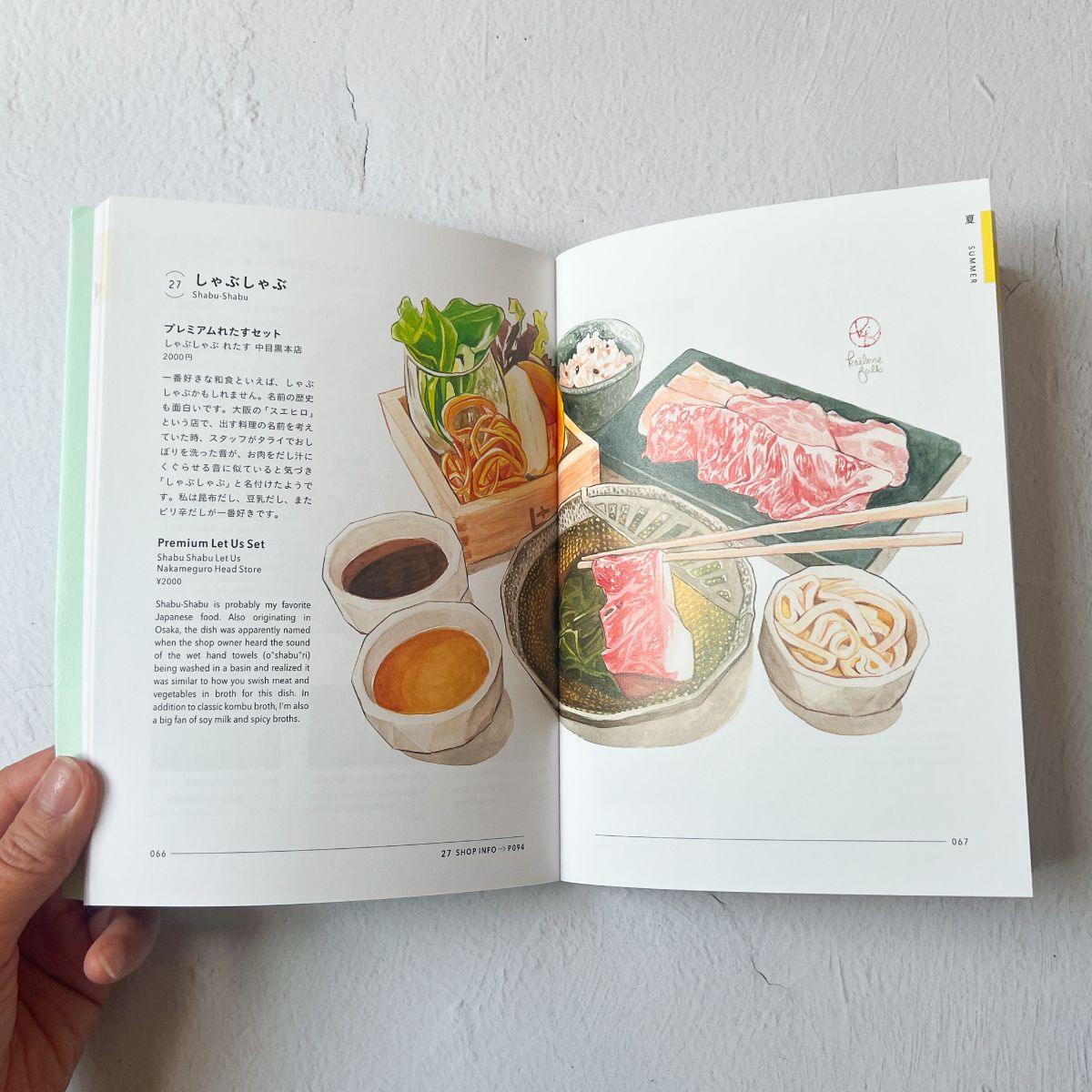This is a close-up, detailed view of a Japanese cookbook open to a specific page. The left side of the page features Japanese text that transitions into English, explaining the history and preparation of "Shabu Shabu," a beloved dish originating from Osaka. The text notes that the name "Shabu Shabu" mimics the sound of swishing meat and vegetables in broth, a key method to this dish, and suggests variations such as kobo broth, soy milk, and spicy broths.

The right side of the page showcases colorful, hand-drawn illustrations of the dish's components and preparation process. The central image is a hot pot containing olive oil with chopsticks dipping a thinly sliced piece of meat into it. Surrounding the pot, the depiction includes a beige cup with onions, two ceramic cups of brown and light brown sauces, a glass holding various vegetables, a half-cut onion, another unnamed orange and red vegetable, a black ceramic bowl with seasoned rice, and a slab holding raw meat.

A portion of a man’s hand is visible at the bottom left, holding the book open. The green cover of the book is partially seen along the left edge. The book rests on or is propped against a rough, white, stucco-like surface, adding texture to the background. This realistic photo captures every detail, from the layout of the food to the precise texture of the paper and background material.